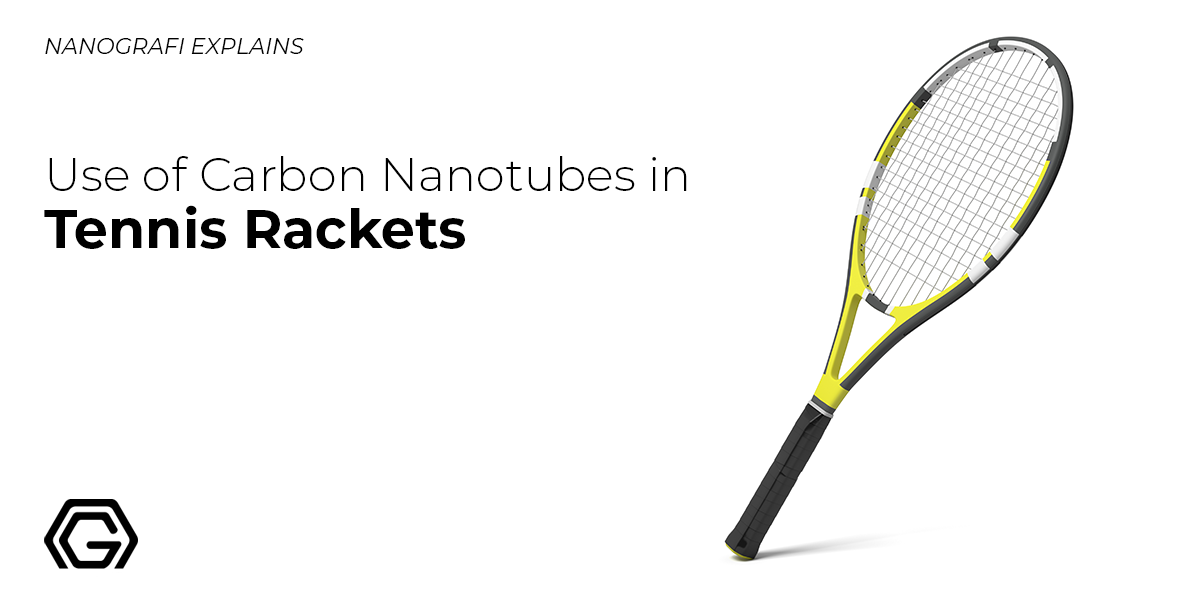The promotional full-color digital image features a sleek, modern tennis racket positioned on the right-hand side against a stark white background. The racket boasts a black handle and a white frame adorned with some striking stripes. On the left-hand side, the text begins at the top in the smallest print, with “NANO GRAFI EXPLAINS” in all capital letters, emphasizing the company name spelled G-R-A-F-I. Below that, in larger letters, it continues, “Use of Carbon Nanotubes in,” leading to a bold and prominent “Tennis Rackets,” positioned centrally. In the lower-left corner, a distinctive six-sided logo with a capital “G” inside marks the branding. The overall layout highlights the advanced materials used in the racket, suggesting a significant enhancement to tennis equipment, as explained by Nano Grafi.